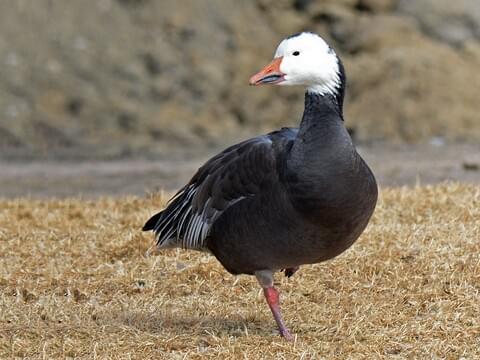This horizontally aligned rectangular picture is a close-up of a medium-sized bird balancing on one leg in the center of the frame. The bird has a distinctive appearance with a white face, small black-beaded eye, and an orange beak. Its head, slightly tilted to the left, transitions from black on the top to the black neck and belly. The wings are black with gray tips and possibly white edges. Only one leg is visible, which is thin and pinkish, adding to its balancing act.

The foreground is filled with dense, dead, brown grass, while the background is a very blurry, rocky, brownish blur that seems to depict the side of a mountain and possibly a road or trail. The outdoor setting gives a natural, slightly rugged appearance to the image.